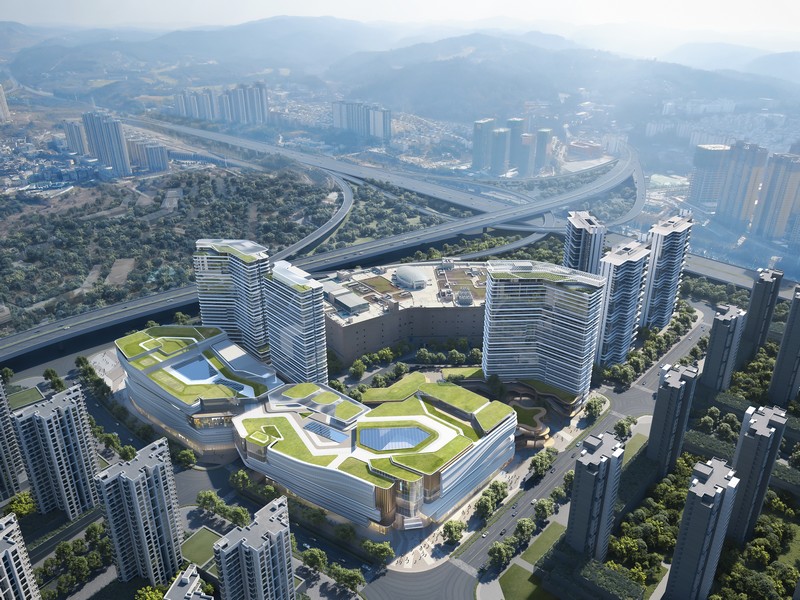This image captures an aerial view of a bustling metropolitan area with a modern architectural landscape. Dominating the foreground, a striking building features an innovative rooftop design with lush grass, water elements, and pathways resembling a golf course, interspersed with trees. Surrounding this building, numerous high-rise structures populate the scene, exhibiting a limited variety of repetitive, rectangular designs, both residential and commercial, with some rooftops potentially housing pools or skylights. Tiny cars and people, resembling ants, crawl along the roads and sidewalks below. The scene extends towards well-traveled roads and a turnpike, eventually merging into tree-lined streets and scattered greenery. Misty, rolling hills and a gray, overcast sky loom in the distance, creating a backdrop of natural beauty contrasted against urban density.